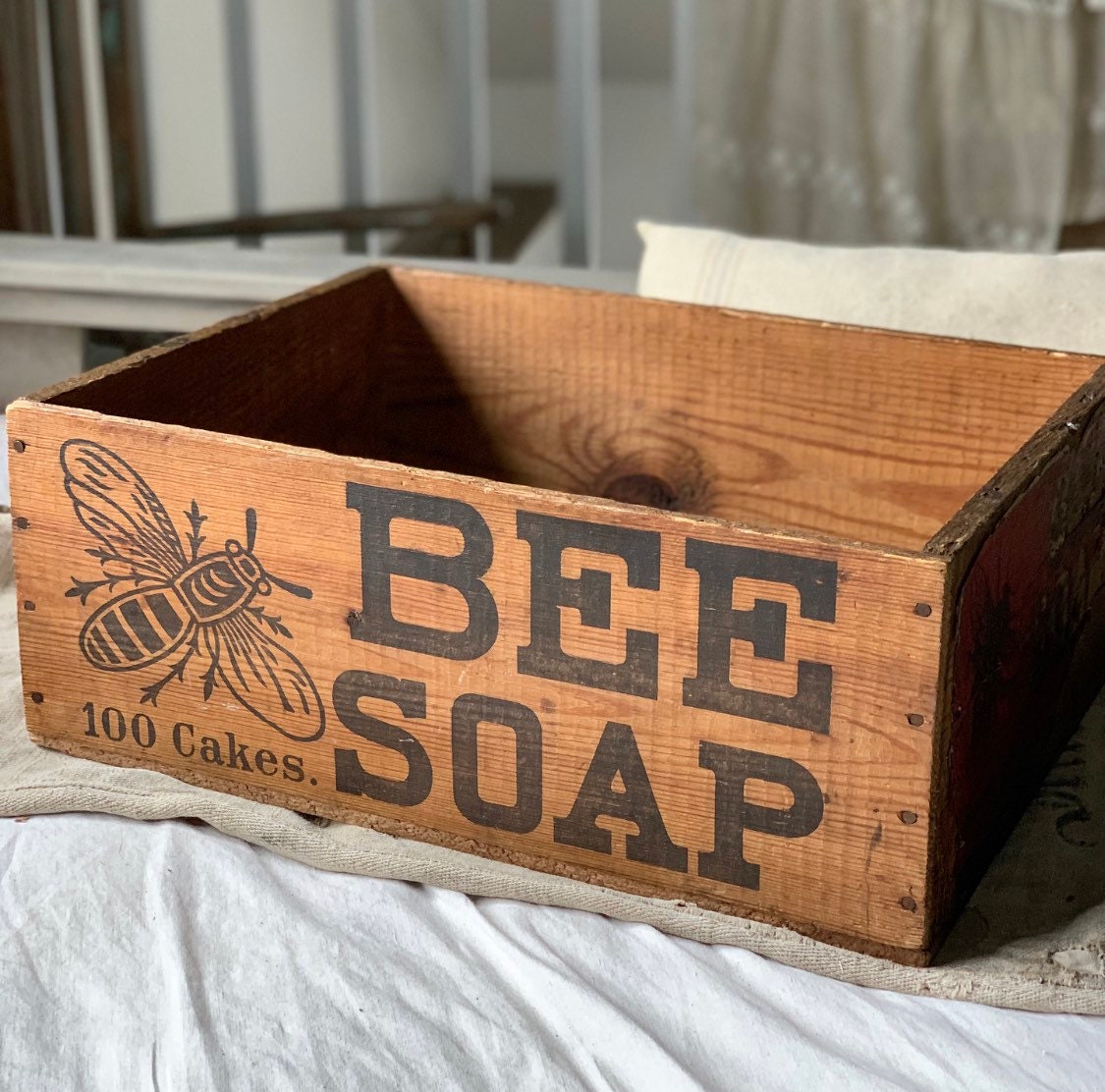This indoor photograph showcases a handcrafted, aged wooden box, exuding a rustic charm with its medium-brown color and prominent dark grain. The shallow rectangular box, visibly fastened together with old nails, prominently features a somewhat faded stencil logo on its front. The left side of the front displays a large black stencil illustration of a bee, beneath which the words "A Hundred Cakes" are inscribed in smaller letters. On the right side, bold black letters spell out "Bee Soap." The box is empty, revealing the raw knots and textures of the wood. It rests on a grayish felt pad atop a white tablecloth or sheet, with a pillow and potentially a railing blurred in the background, suggesting a cozy indoor environment.